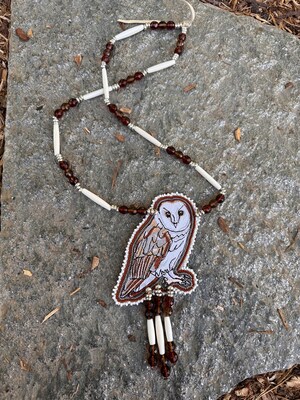In this image, we see a distinctive necklace prominently displayed on a gray, rocky surface outdoors, surrounded by hints of crushed brown leaves and patches of grass. The necklace features an intricate owl pendant with an array of colors in its wings and a slightly fierce expression. The owl, primarily white or silver with a red outline, is accented with beads that are brown and white. The pendant is complemented by three beaded strands hanging below it, alternating between the brown and white hues. The necklace itself consists of a series of longer brown beads interspersed with clusters of smaller beads. This artistic piece, evoking a deep connection to nature, appears perfectly at home in the sunlight against the natural stone backdrop.